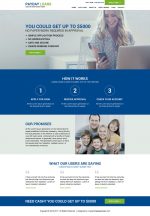This image is an extremely blurry screenshot of a webpage. The top one inch of the page is white, followed by approximately three inches of light gray background. Beneath this light gray section, there is a dark blue strip about two inches high, which transitions back to light gray and then returns to white for around two inches before reaching another dark blue section at the bottom of the page.

At the top left corner, there is some indiscernible blue lettering, followed by additional illegible text underneath. On the right side, the page features six tabs with black text that cannot be clearly read. Above these tabs, there is a green tab with white lettering. In the light gray section below, a blonde-haired woman is pictured looking down at her phone. To her right, a laptop is visible, and above it, part of the text reads, “you could get up to 15,000 maybe.” Below this, there is black text and four bullet points, each accompanied by its own text. Another green tab with white lettering is positioned underneath this section.

In the dark blue section, the terms “how it works” are visible, followed by the numbers one, two, and three each enclosed in gray circles. There is more text below these numbers. In the next light gray area, there is an image of a family consisting of a man, his wife, a little girl, and two boys, with a paragraph of text beside them. Underneath this, the page returns to white, bearing some text that is partially discernible as “what our Liberty ...”, followed by three rows of additional text. The bottom section of the page is dark blue with white lettering, and a green tab is located on the right side.